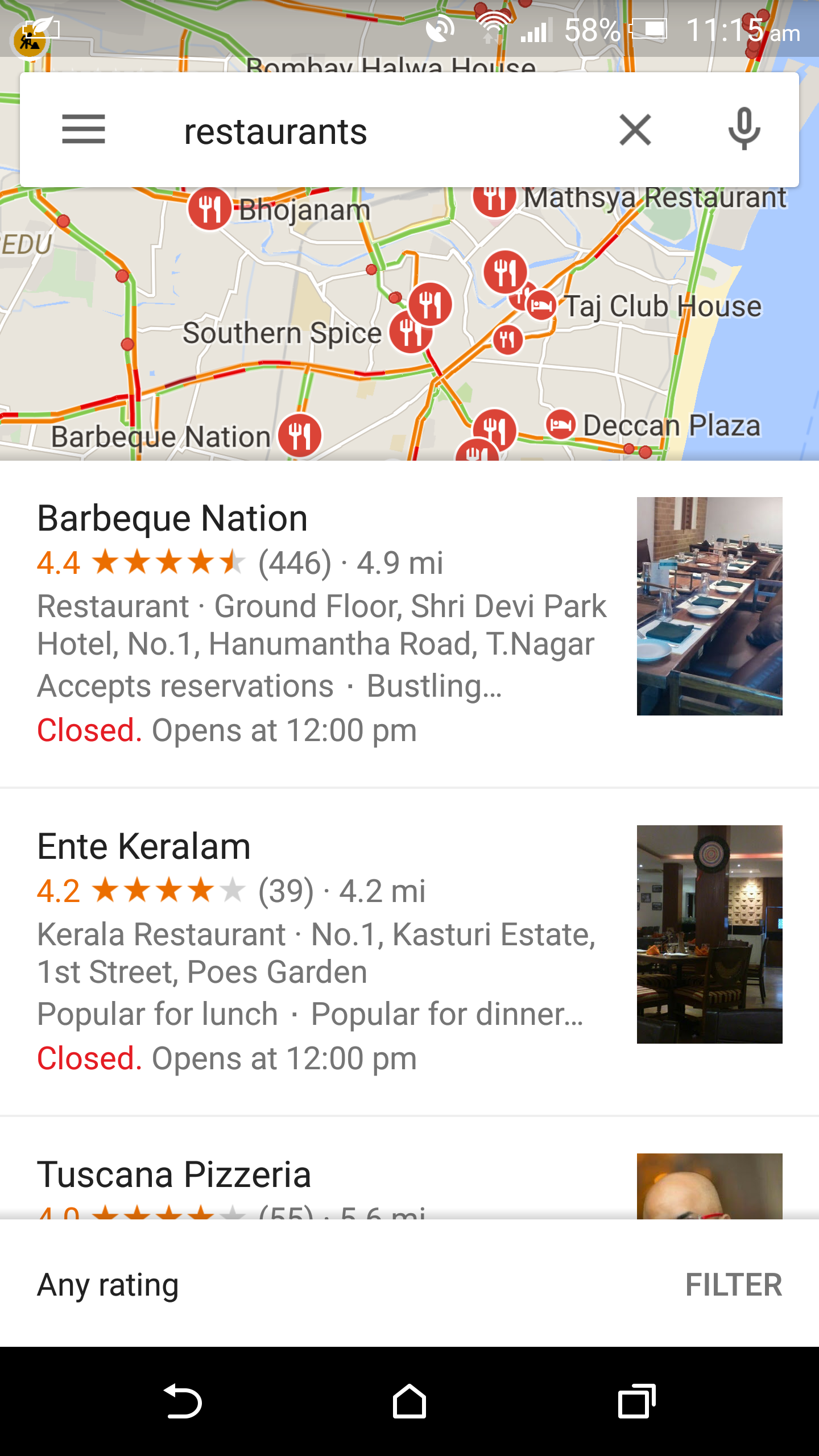The image displays a detailed map highlighting various restaurant locations. Key establishments featured include:

1. **BBQ Nation**, rated 4.4 out of 5 stars based on 446 reviews. This restaurant is located 4.9 miles away and can be found on the ground floor of the Sreedevi Park Hotel at No. 1 Martha Road, T. Nagar. BBQ Nation accepts reservations and is currently closed, with an opening time of 12 PM.
   
2. **Antique Carillon**, rated 4.2 out of 5 stars from 39 reviews, situated 4.2 miles away at 1st Street, Fool's Garden. This restaurant is popular for both lunch and dinner, is currently closed, and also opens at 12 PM.

Other notable locations marked on the map include Deccan Plaza, Taj Clubhouse, Southern Spice, Boba John's, and Matheson Restaurants.